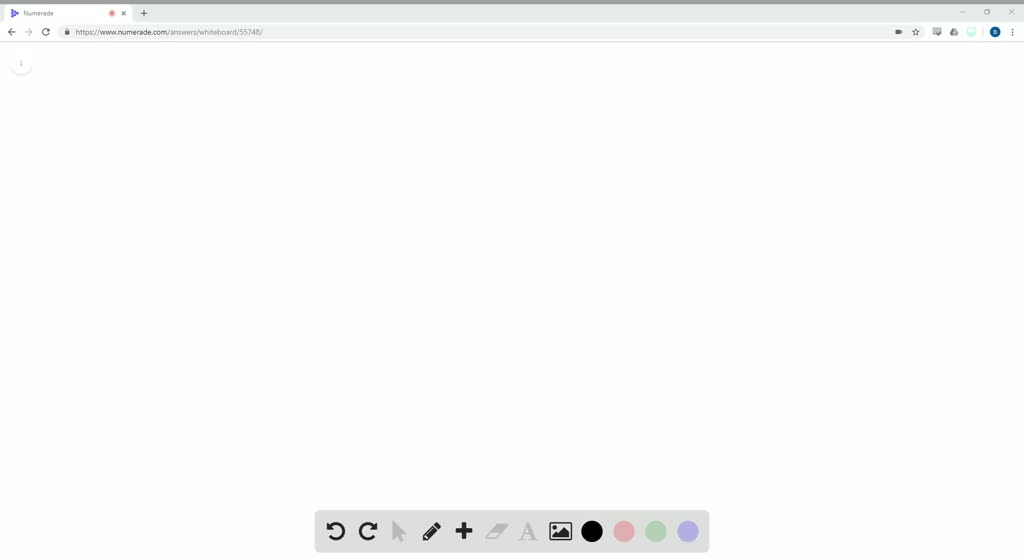A detailed screenshot of the blank interactive whiteboard on the website NUMERADE.com/answers/whiteboard/55748. The interface, designed as a versatile canvas, is primarily blank, offering users the creative freedom to draw and annotate. At the bottom of the page, a toolbar provides various options for customization and interaction. These include buttons for drawing shapes, inserting images, undoing and redoing actions, arrows, and a selection tool. Users can choose from pens or markers for drawing, and a plus sign likely for adding new elements. Additional options include an eraser, a font icon for text, and a picture icon for embedding images. The toolbar offers a palette of four colors: black, pink, light green, and purple, to enhance the visual creativity.